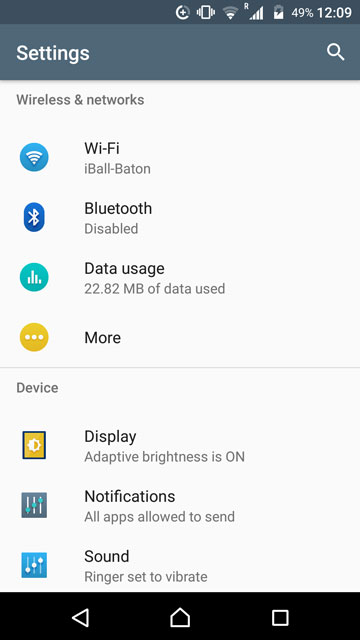This screenshot from a phone captures multiple UI elements, all meticulously arranged for user clarity. At the very top, there's a dark gray status bar featuring essential phone icons: a Wi-Fi signal, cellular signal bars, a battery indicator at 49%, and the current time displayed as 12:09. Below the status bar lies a lighter gray section, segmented to enhance readability. On the left, prominently displayed, is the word "Settings," while to the right, a magifying glass icon denotes the search function.

The main content area beneath this section is set against a crisp white background. It starts with the header "Wireless and Network," followed by several key options listed in a vertical format. First among these is "Wi-Fi," with the network name "Eyeball-Baton" indicated next to it. Following this, "Bluetooth" is shown as "Disabled," accompanied by the Bluetooth logo. Further down, "Data Usage" is detailed, showing "22.82 MB of data used." Below this, a yellow circle featuring an ellipsis hints at additional options, labeled succinctly as "More," with a light gray dividing line below it.

The next category is "Device," offering a quick overview of several settings. "Display" indicates that "Adaptive Brightness is On." "Notification" follows, detailing that "All Apps Allow to Send" notifications. Lastly, "Sound" is noted, showing that the "Ringer Set to Vibrate."